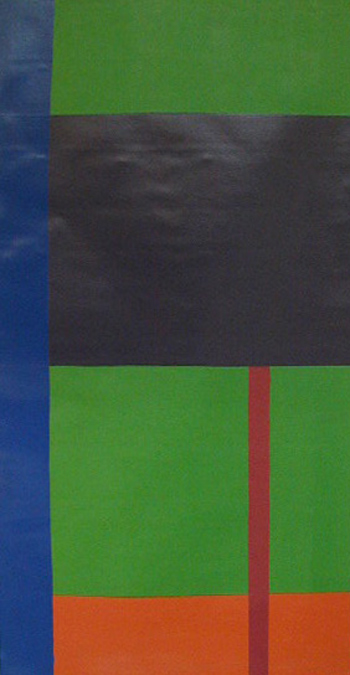This is an abstract, cubist-style painting characterized by a series of simple shapes and minimal use of color. The artwork is a long, rectangular piece, approximately three to four feet in length and one and a half feet wide. Dominating the left side of the composition is a thin, vertical navy blue stripe that runs the full height of the canvas. To the right, the painting is divided into a series of stacked rectangles and squares in varying colors.

At the top of the right side is a forest green rectangle, followed by a larger black rectangle beneath it. Below the black rectangle is another green shape, this time a square, followed by an orange rectangle at the bottom of the stack. A thin red stripe intersects both the green and orange sections horizontally, adding a dynamic element to the otherwise vertically oriented shapes. The black square is notably connected to a darker crimson red stripe.

The painting features a bit of texture, with visible bumps and ripples, suggesting that parts of it might have been created using tape, particularly around the blue stripe. The composition's simplicity and geometric form evoke a cubist aesthetic, emphasizing the contrast between the colors and the shapes.